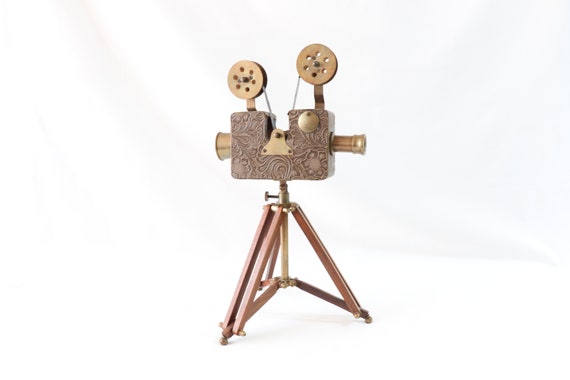In the image, there is an intricately designed old-fashioned movie camera mounted on an adjustable, collapsible tripod. The tripod is crafted from brass and wood, radiating an antique charm. The camera itself, turned slightly to the side, is adorned with ornate floral designs in relief and is predominantly a mauve or light brown color. Both sides of the camera have brass elements; the left side features a brass decorative piece, while the right side has a broader brass viewing tube resembling an old spyglass for the person filming. On the top of the camera, two brass film reels with holes are mounted, with what appears to be film running between them, creating a graceful dip in the center. The entire apparatus is set against a mostly white background with subtle light gray accents, emphasizing the detailed craftsmanship and nostalgic aesthetic of this apparent artwork.